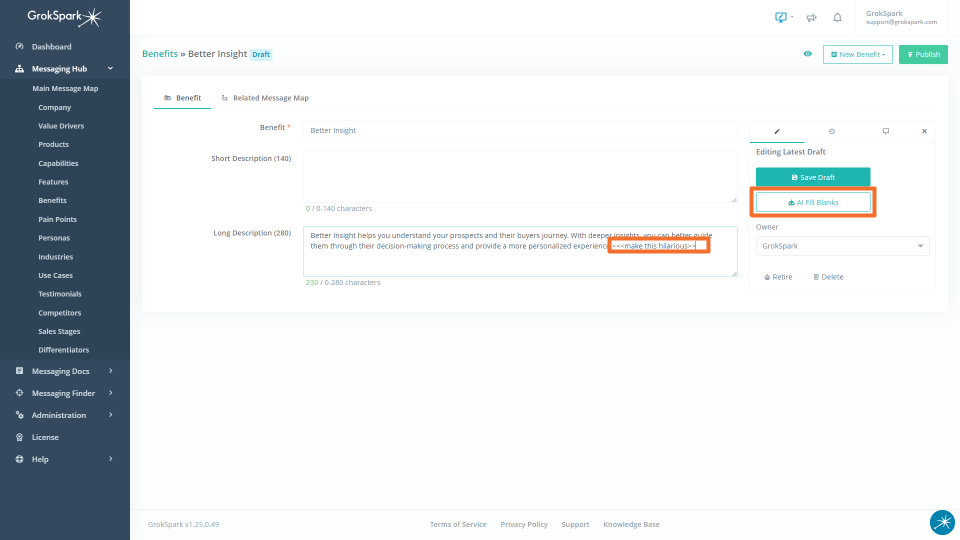The image depicts a user interface from a software called GrokSpark. On the right-hand side, a dark teal rectangle spans the full height of the screen. At the top of this rectangle, the word "GrokSpark" is prominently displayed in white, accompanied by an icon resembling a scepter with a sparkle. Below it, also in white, are the words "Dashboard," "Message," and "Hub."

Further down, a series of terms appear in white text: "Main Message Map," "Company," "Value Drivers," "Products," "Capabilities," "Features," "Benefits," "Pain Points," "Personas," "Industries," "Use Cases," "Testimonials," "Competitors," "Sales Stages," "Differentiators," "Message Inducts," "Messages Finder," "Administration," "License," and "Help."

The primary background transitions to a very light gray, almost off-white color. At the top left of this section, the word "Benefits" is highlighted in green. Adjacent to this, two gray rectangles and a black rectangle delineate sections, with the black one labeled "Better Insight."

On the same horizontal line, a dark blue rectangle with the label "Draft" precedes two smaller rectangles. One is white with a green outline and labeled "New Benefit," while the other is green with a white outline and the word "Publish."

Above this row, in gray text, "GrokSpark" is followed by "Add support" and "support@grokspark.com."

In the subsequent row, where the background turns white, the words "Benefit" (underlined in green), "Related," and "Message Map" appear in black. A thin line runs horizontally across the screen, followed by sections labeled "Better Insight," "Benefit," "Short Description," and "Long Description."